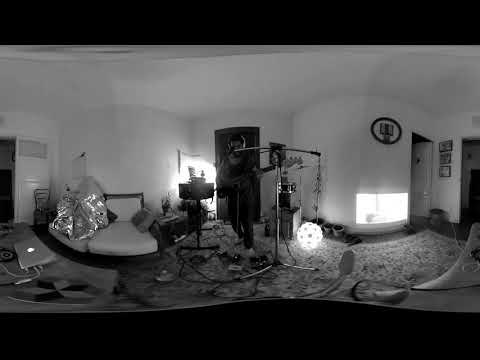This black-and-white photograph captures a musician performing in what appears to be a recording setup within a residential space, potentially a living room or bedroom. The shot, taken with a wide-angle lens, centers a man dressed in black playing a guitar with a microphone on a stand positioned before him. He stands against a backdrop of predominantly white walls, flanked by a doorway directly behind him and another to his right. To the left side of the image, a bed or possibly a sofa is visible, characterized by what seems to be a distorted or curved effect due to the lens. Additionally, a cell phone can be seen charging on a nearby dresser, accentuating the room's casual, lived-in atmosphere. The floor features an intricately patterned, likely Asian-style rug, upon which various electronic devices are scattered, suggesting a home recording environment. Notably, a white, spiky, glowing orb rests on the floor near the center to the right of the performer, adding an unconventional, intriguing element to the scene. The left side of the room also showcases a large, lumpy piece of silver foil adorned with a whimsical monster face drawing, juxtaposing humor with the more serious musical endeavor. Further details include several flower pots, three framed pictures on the walls to the right, and what could be a fireplace, anchoring the setting in a comfortably creative space.